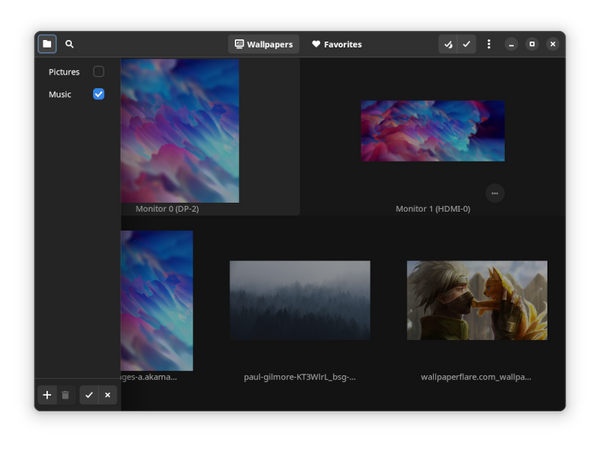The image depicts a digital interface on a black screen with various elements laid out primarily in white. On the left side, there is a file icon followed by a search menu. Below these, the words "Wallpapers and Favorites" are displayed, accompanied by a heart icon. Adjacent to these are two check marks. Further down, there are three vertical dots, typically indicative of more options. The interface also includes standard window operation icons for closing, minimizing, and maximizing the screen.

Additionally, the screen displays two sections labeled "Pictures" and "Music," the latter marked with a blue check mark. Beneath these labels, a visual thumbnail or icon of a monitor is shown with the text "Monitor 0 dp-2" and next to it, "Monitor 1 hdmi 0," alongside three dots arranged in a circular formation.

At the bottom of the screen, the following text is visible: "images a.akama," "paul-bilmorekt3wlrl_bsg_," and "wallpaperflare.com_wallpaper." 

On the extreme lower-left corner, there is a plus sign, a recycling bin icon with a check mark next to it, and an 'X' symbol. 

Overall, the image is a detailed screenshot of a file management or image browsing interface with various organizational and navigational elements.